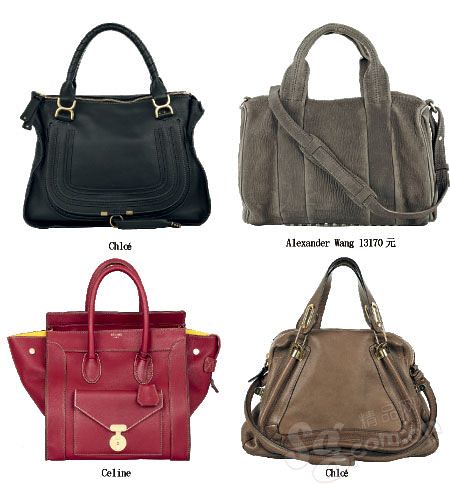The photo depicts four women's purses arranged on a white background, each labeled with brand names beneath them. 

The top left purse is a black leather Chloe bag with a steel clasp on the handle and silver buckles. To its right is a gray suede-like Alexander Wang bag, which features a gray strap across the middle and the number 13170 with Japanese characters next to it. Below the black Chloe purse, in the bottom left corner, is a red leather Celine bag. This bag has a yellow accent, red pockets extending from the sides, a red handle going over the top, and a silver buckle at the front. To the right of the red Celine bag is a light brown or beige Chloe purse with rugged detailing, gold buckles attached to the clips at the top, and a larger strap extending across the middle.